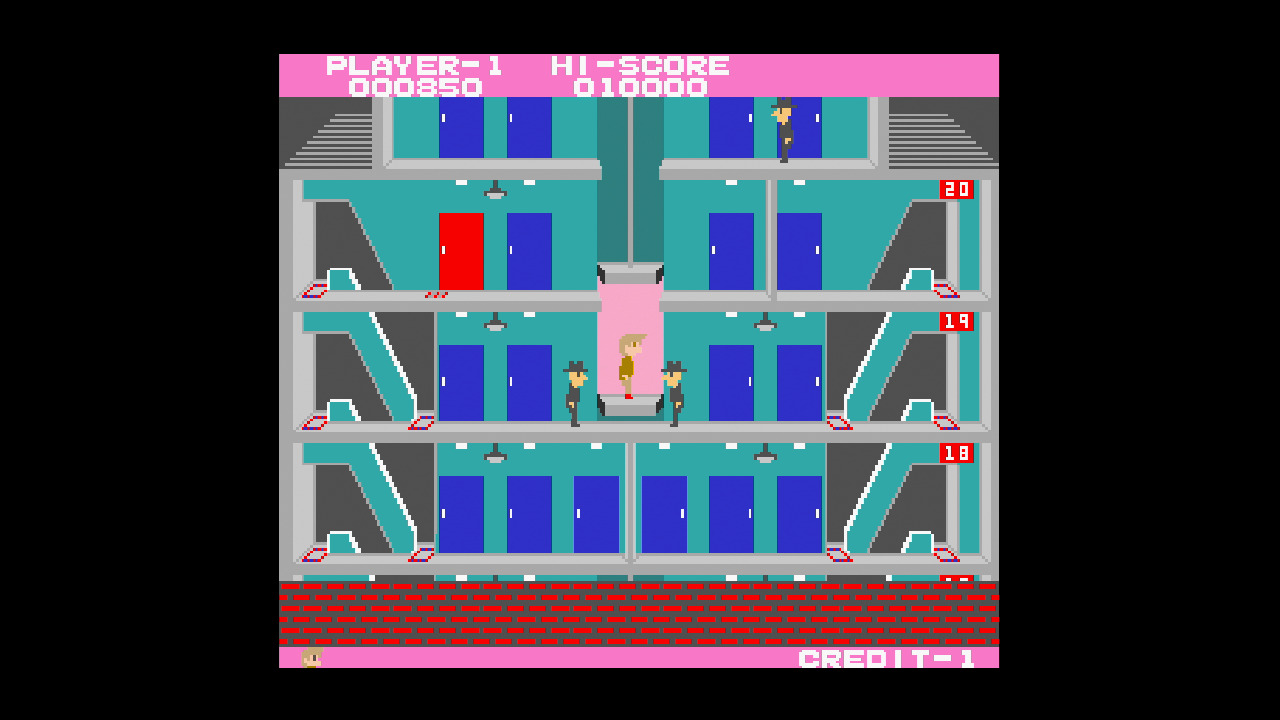This image depicts a detailed screenshot from a retro-style video game, reminiscent of a Cops and Robbers theme. The gameplay involves navigating multiple floors connected by blue doors and a central elevator that moves vertically. The setting features a teal background with elements such as a wall at the bottom adorned with red bricks. 

The action centers around an elevator where one character is enclosed, with two additional characters positioned as if prepared to intercept. On the top right corner of the screen, another character, likely a cop, is visible, intensifying the chase dynamic. The scene includes several numbered floors, specifically 18, 19, and 20, and various blue and red doors spread across the middle and lower sections. 

Key interface elements are highlighted by pink banners: on the top left, "Player 1" score is listed as 850, while the high score proudly displays 10,000. Additionally, a "Credit 1" indicator in the bottom right corner suggests it’s a single-player game. The visual style features pixelated little figurines, amplifying the nostalgic feel of the game. The ultimate goal appears to be maneuvering between different floors to achieve a high score, navigating through numerous obstacles and characters.